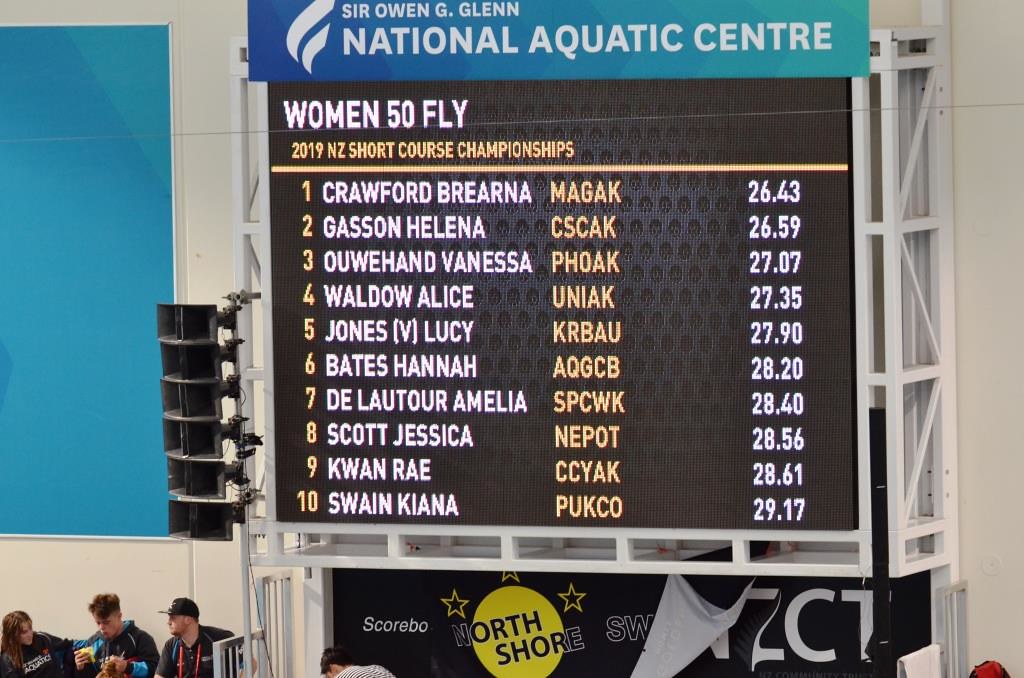The image depicts a detailed scoreboard at the Sir Owen G. Glenn National Aquatic Center, showcasing the results of the Women 50 Fly event from the 2019 NZ Short Course Championships. Dominating the scene is the turquoise-hued scoreboard, listing the top 10 competitors and their respective times. At the top of the list is Crawford Browna with a time of 26.43, followed by Gasson Helena at 26.59, and Ohand Vanessa at 27.07, extending to Swain Kiana, who clocked in at 29.17. Beneath the primary information on the board, an advertisement for North Shore is partially visible, with the banner appearing slightly detached. To the left of the scoreboard, a stack of speakers is positioned above three spectators seated in bleachers, attentively watching the championships unfold.